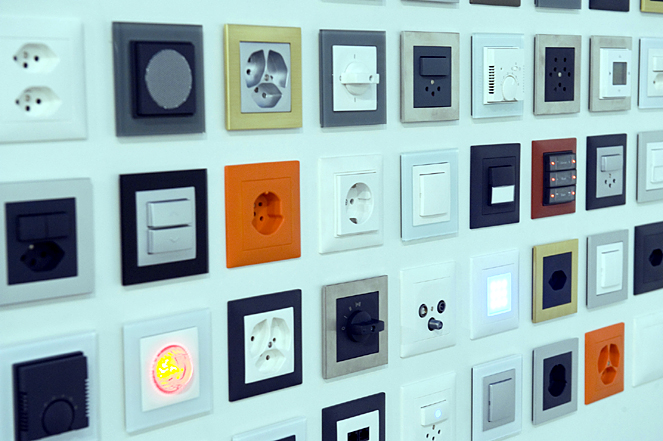This color photograph captures a close-up of an intriguing art installation featuring a series of lined-up squares, possibly framed panels, mounted on a white wall with a cyan tint. These panels, organized in neat diagonal rows from the left-hand portion to the right-hand portion of the image, display a variety of different types of outlets, switches, sockets, and other wall inserts. The collection includes a diversity of colors and styles, representing different countries. Predominantly, the panels are shades of white, navy blue, orange, black, khaki, silver, and red. Notably, there are several lit elements: a bright light in one square with pink around the outside and yellow inside, located at the bottom left; an orange and red light also at the bottom left; red switch lights in the right middle section; and a thermometer towards the top right. Additionally, there is a telephone jack or internet cable connector situated in the center bottom right. The vivid hues and varied textures make this installation a vibrant and multi-faceted visual experience.